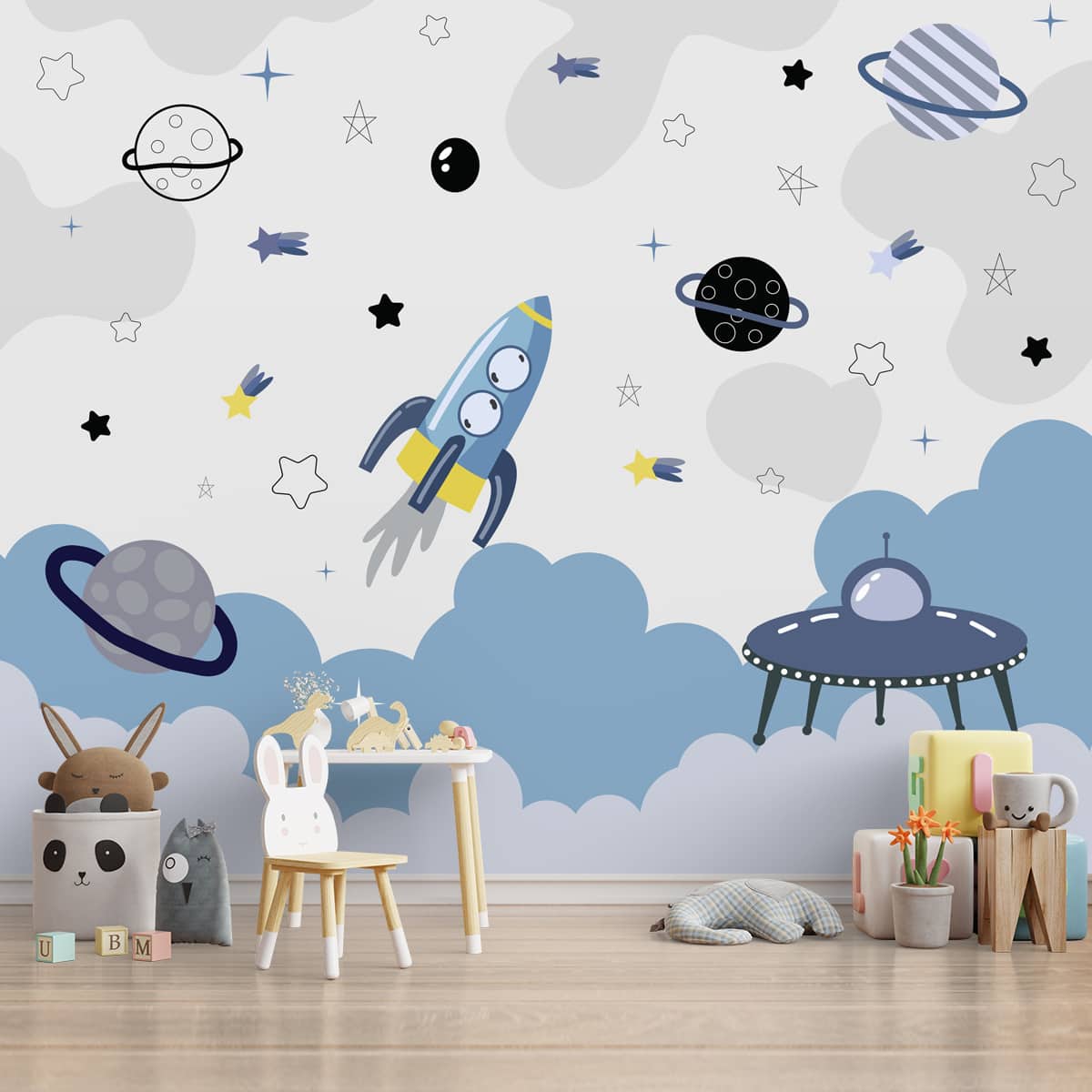This professionally taken color photograph features a meticulously decorated children's room or nursery. The prominent mural on the wall depicts an outer space theme with a light blue rocket ship front and center, surrounded by various planets—some with rings—along with stars, shooting stars, clouds, and two additional spacecraft, one of which is a UFO. The mural vibrantly combines shades of gray and blue against a cream-colored background, creating a whimsical yet serene scene. The room is well-lit, showcasing a light brown, shiny wooden floor.

In the foreground, a small children's table is accompanied by a charming chair with a bunny face backrest and ears. Scattered across the floor are various playthings including plush toys—a stuffed rabbit and owl—a basket resembling a panda, and a pot of orange flowers. Wooden blocks with pastel colors, prominently showing the letters "UBM," add a playful touch, alongside larger foam blocks, a smiling face cup, and a toy potted plant with flowers. The meticulously arranged objects and clean studio setting underscore the room's purpose as a child’s playful sanctuary.